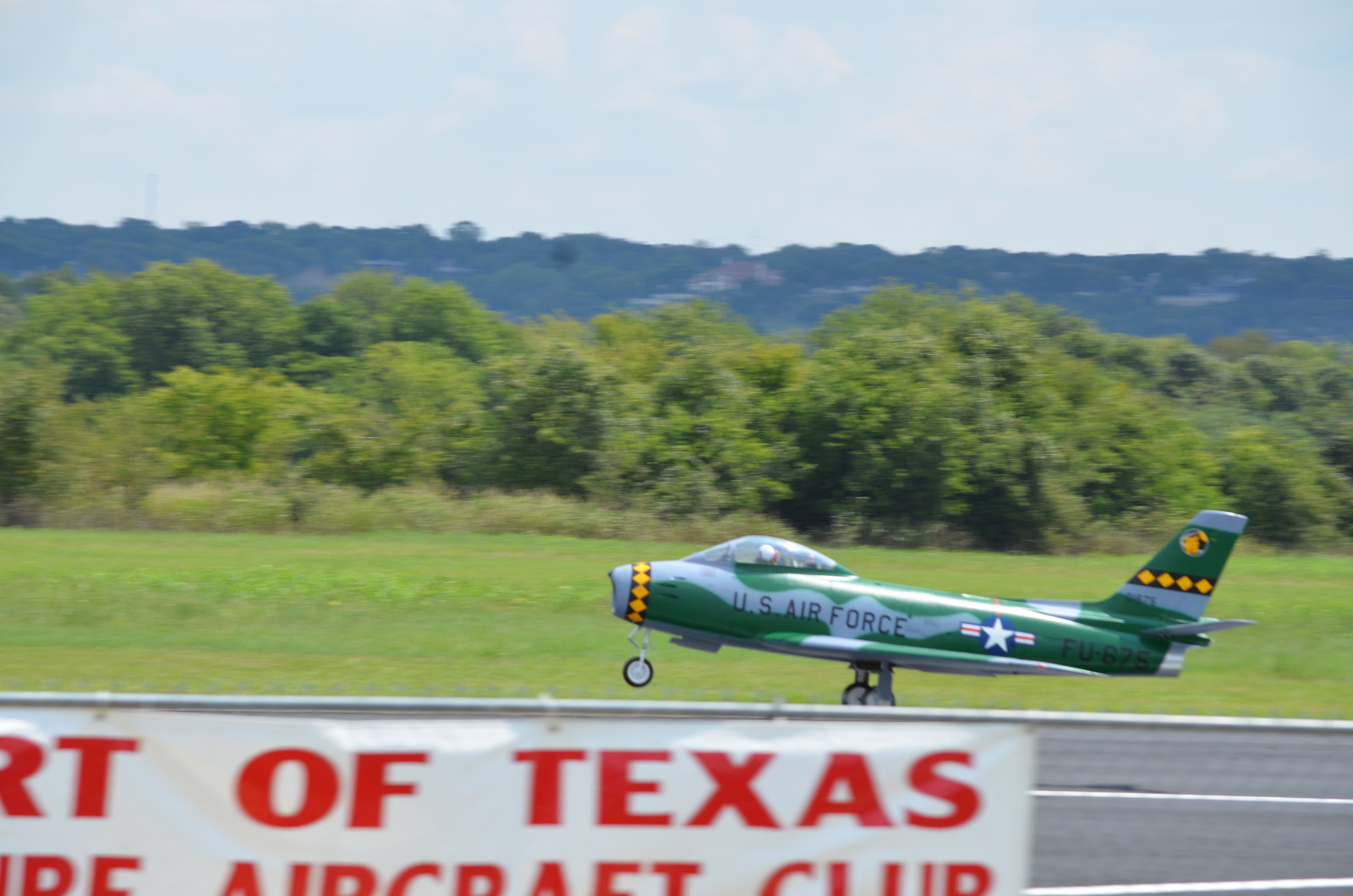This detailed outdoor photograph showcases a lively airfield during the day. At the bottom right of the image, an asphalt pavement transitions into a grassy field, bordered by trees and bushes. Just above the runway, central to the image, a United States Air Force aircraft, painted green with blue text, "U.S. Air Force," and bearing the number "FU875," is seen taking off. The pilot is visible in the cockpit. In the foreground, there's a fence with a partially visible banner reading "R.T. of Texas" and likely "Aircraft Club" in red text. The background reveals an expansive green field, sloping up to a horizon lined with trees and buildings, under a clear blue sky. The color palette includes shades of light blue, white, gray, green, dark green, yellow, brown, red, and gray, indicating a bright, midday setting at a small airport.